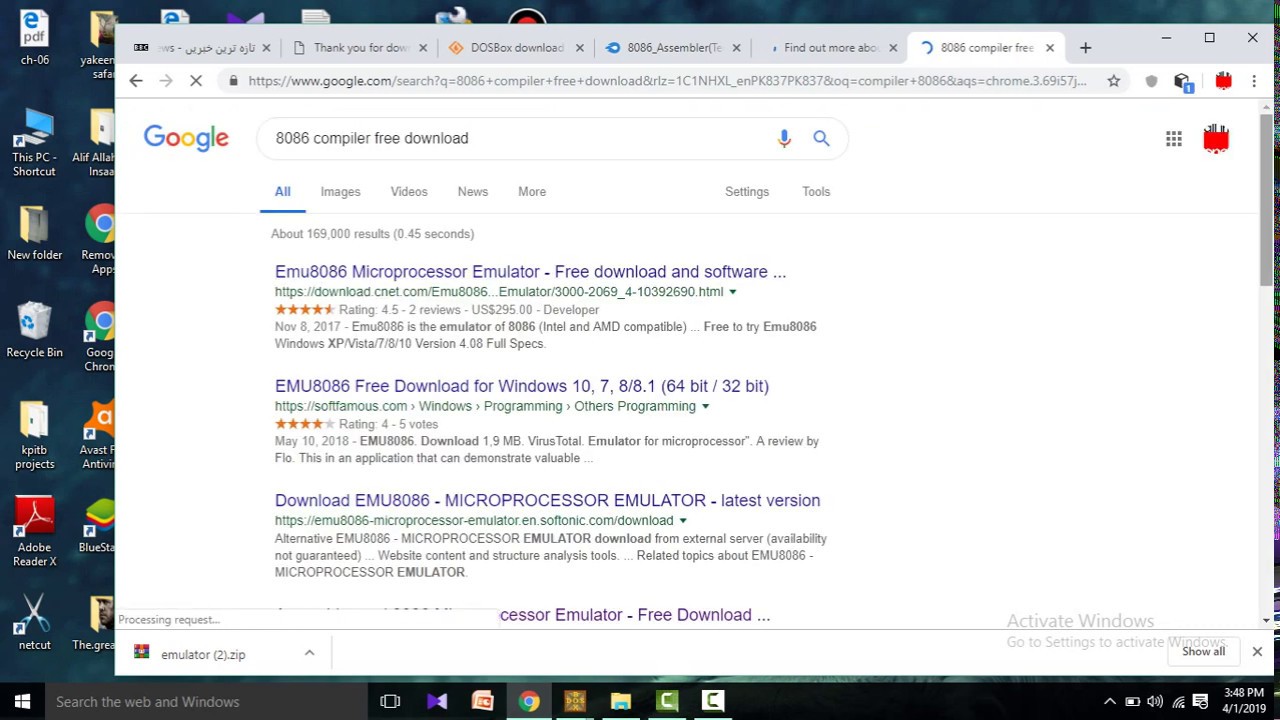A screenshot depicts a computer screen with a web browser occupying approximately 80% of the visible area. The browser has six open tabs, and the URL in the address bar reveals a search query for "Google 8086 compiler free download." The search results page includes sections for images, videos, news, more, settings, and tools, with "all" underlined in blue to indicate the selected category. The search has yielded about 169,000 results in 0.45 seconds. Prominently featured among the search results is a listing for the EMU8086 microprocessor emulator, which boasts a high rating of four and a half stars based on two reviews. Another result highlights the availability of EMU8086 for free download on various Windows operating systems, including Windows 10, 7, and 8/8.1, compatible with both 64-bit and 32-bit architectures, and features a rating of four stars based on five votes. The list also advertises the latest versions of the EMU8086 microprocessor emulator, which is capitalized for emphasis.